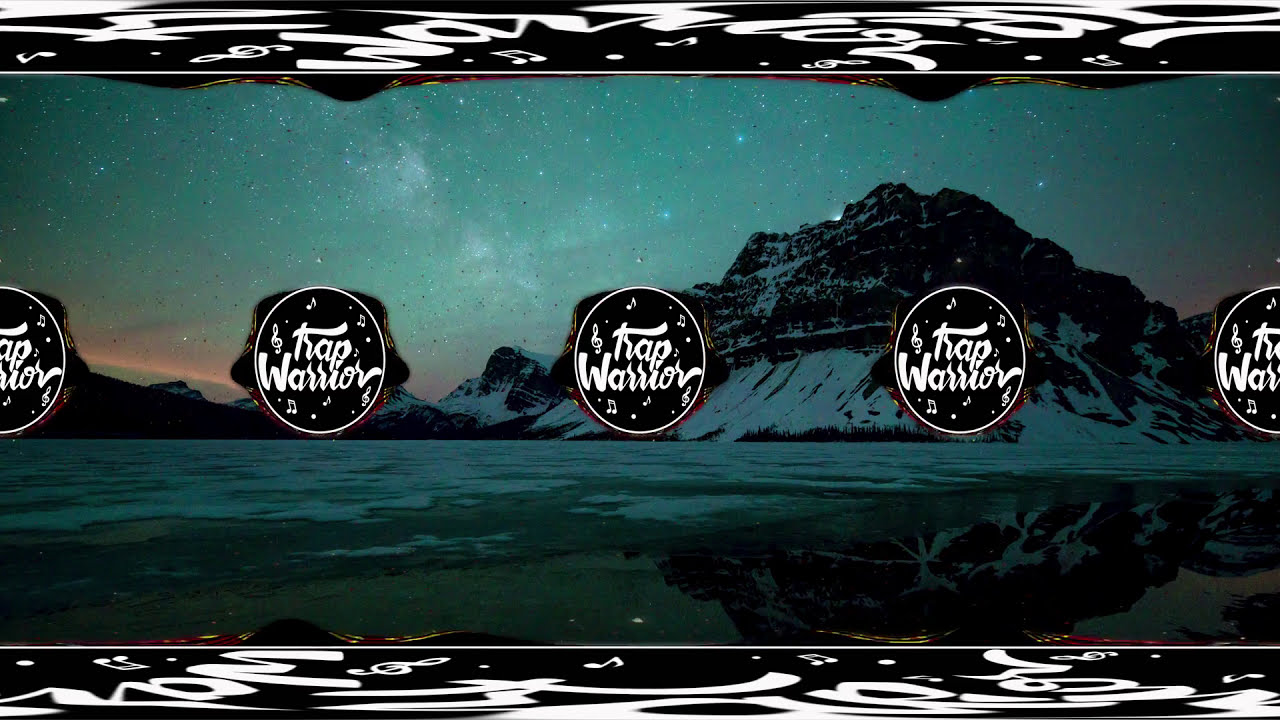This graphic advertisement for "Trap Warrior" or "Hop Warrior" features a striking mountain scene set against a star-studded evening or nighttime sky. The landscape is bathed in muted teal green, white, and hints of pink, presumably from a setting sun, giving it an overall bluish-white appearance. The serene mountain is mirrored perfectly in a frozen lake below, adding to the cold, tranquil atmosphere. Central to the image are five circles arranged horizontally; three full circles span the center, flanked by two half circles at the edges. Each circle is black with a white rim and contains white text that reads "Trap Warrior" along with musical notes. Identical black bars with white graphics line the top and bottom of the image, adding symmetry. This carefully designed scene captures a fusion of natural beauty and musical branding.